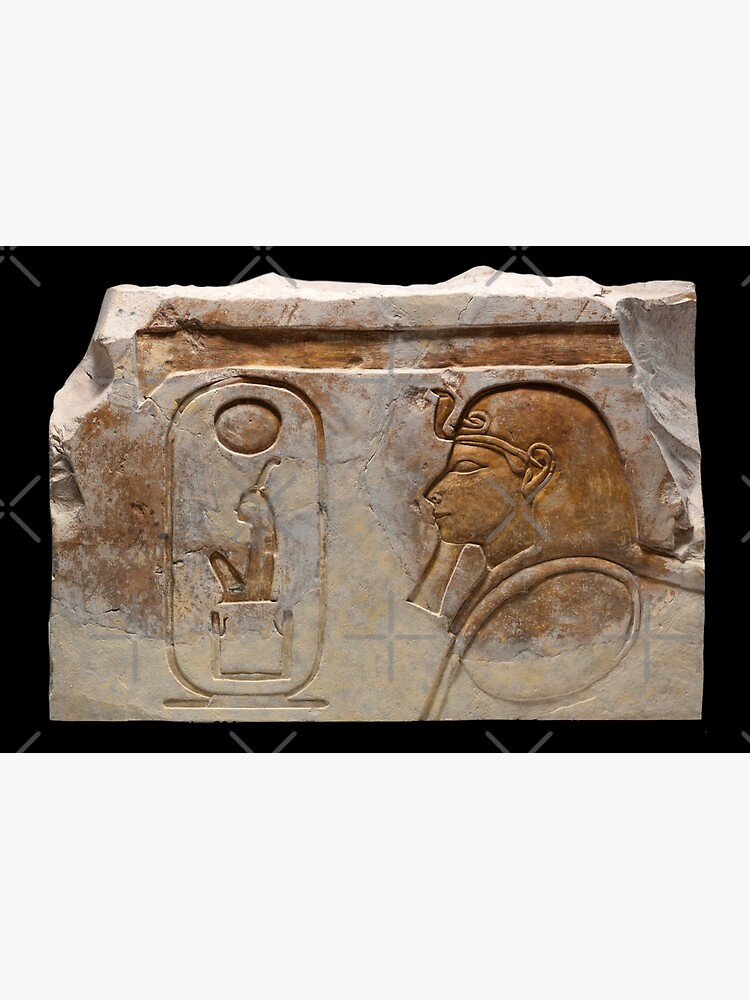This photograph showcases an ancient Egyptian artifact, likely a fragment of a larger stone relief, set against a stark black background. The beige-brown stone features two distinct carvings and exhibits ragged edges, suggesting it was once part of a wall or larger piece. On the right side, there is a detailed profile of a figure resembling a young pharaoh, possibly designed in a caricature style. The pharaoh's head is adorned with a headdress that includes a cobra emerging from the forehead, indicative of royal status, and a long beard trailing from the chin. The face, shoulder, and ear are clearly delineated. On the left side, the artifact presents an oval-shaped cartouche, a traditional Egyptian hieroglyphic element often containing a name. Within this cartouche, a small figure appears seated with knees up, surmounted by a vertical line and floating above two smaller figures with uplifted arms, possibly supporting the seated figure. At the top of the cartouche, a large circle, possibly representing the sun, is depicted. The artifact is marked with a gray, crosshatched watermark that includes pluses and Xs across the photograph, suggesting it is a protected image. The overall condition and intricate details of the stone carvings confirm its ancient origins and cultural significance.